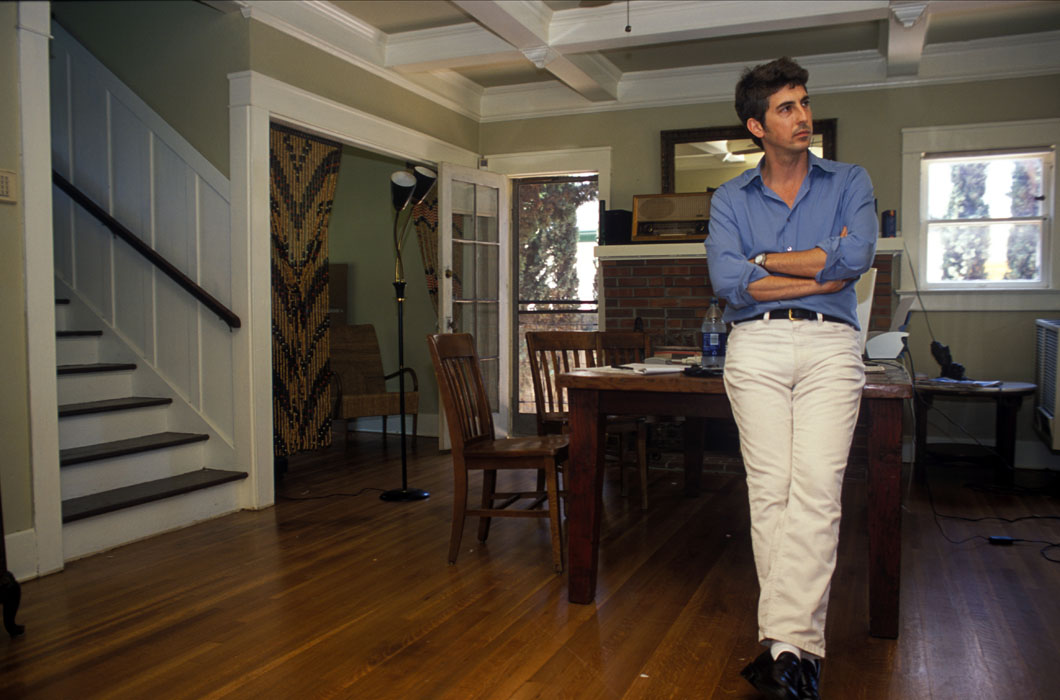In the photograph, a man is positioned on the right side of the living room, leaning against a large wooden table with his legs crossed and seated on its edge. He is dressed in white jeans with a black belt and gold buckle, black leather dress shoes with white socks, and a blue button-up long-sleeve shirt with the sleeves rolled up to his elbows, revealing a silver wristwatch. His dark brown hair is styled neatly, and his face is turned towards the top right of the frame while his body faces forward. Scattered across the wooden table are a plastic water bottle with a blue label, multiple sheets of paper, a computer, and a stand-alone printer. Wooden chairs are aligned along one side of the table. The room features wooden flooring, a red brick fireplace behind the table, and a white staircase leading upstairs to the right. Various wires and extension cords are visible on the floor. A door leading outside stands open to the right of the fireplace, and a window is positioned to its left, offering a glimpse of trees outside. The walls appear to be a light brownish green shade.